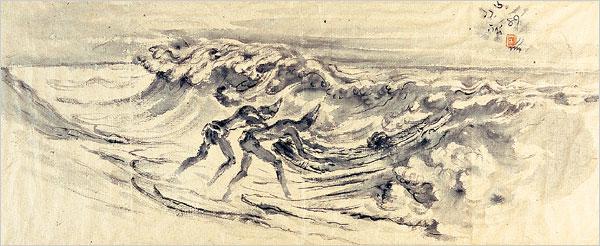This horizontal, rectangular drawing features a grayscale palette with subtle accents of light pink and orange, making it an evocative piece of artwork. The scene is set outdoors, capturing a dramatic moment by the ocean. The sky, depicted with swirls of gray and white, transitions to a slightly pink hue near the top with fluffy clouds scattered across it, and there's a hint of yellow in the upper right corner that might depict a bird. Below, the landscape slopes downward on the left, resembling a hill or sandy shore. Central to the image are two thinly drawn figures, who appear to be Indigenous men wearing conically shaped hats, possibly ceremonial, with small feathers hanging from their waists. Positioned in the midst of high, choppy waves, these men are bent over, pushing a canoe with extended arms against the rushing waters. The waves are rendered in dark gray tones with white crests, adding to the tumultuous atmosphere of the scene. There is no text present in this hand-drawn, low-quality sketch, leaving the focus solely on the interaction between the men and the powerful ocean waves.